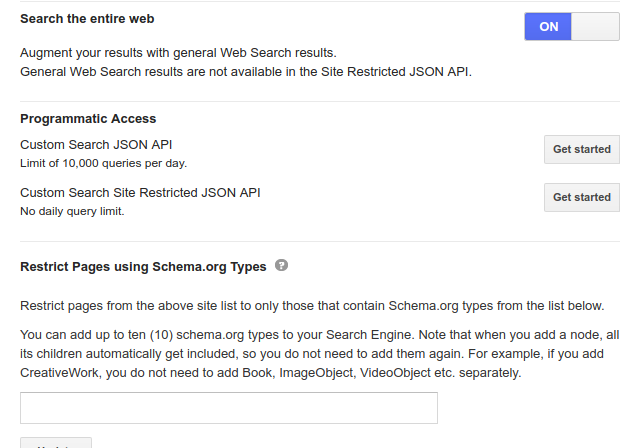The image displays a web page with a clean, white background and black text for easy readability. At the top of the page, there is a prominently bolded header in dark black that reads, "Search the entire web." Below this header, there is an informational text stating, "Augment your results with general web search results. General web search results are not available in the site-restricted JSON API." Adjacent to this information is a toggle button that can be turned on or off. The button is blue with white text and is currently in the "On" position.

Further down, another dark black bolded section titled "Programmic Access" is featured. Beneath this title, it specifies, "Custom Search JSON API limit of 10,000 queries per day," with a "Get Started" button positioned to the right. Following this, the page notes, "Custom Search Site-Restricted JSON API," and adds that there is "No daily query limit." Accompanying this text is another "Get Started" button to the right.

The next section, also in bold, labeled, "Restrict pages using schema.org types," includes an interactive question mark button for additional information. Below this, the page explains, "Restrict pages from the above site to list only those that contain schema.org types from the list below. You can add up to 10 schema.org types to your search engine. Note that when you add a node, all its children automatically get included. So you do not need to add them again. For example, if you add CreativeWork, you do not need to add Book, ImageObject, VideoObject, etc., separately."

At the bottom of the page, there is a text box for users to add their desired schema.org types to further customize their search engine.